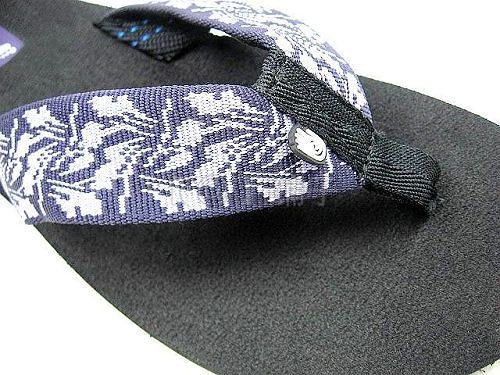This color photograph features a close-up view of a single flip-flop, oriented diagonally with the back of the shoe in the upper left-hand corner and the toe area in the lower right-hand corner. The flip-flop has a black textured sole, upon which sits a Y-shaped strap. The centerpiece of the strap, which fits between the toes, is constructed from black fabric. 

The straps themselves are purple with intricate white abstract designs, resembling flowers. These straps extend from the sides across the top of the foot, creating a secure hold. Distinguishing turquoise (light blue) double stitching is visible where the straps are sewn into the sole, adding a pop of color and detail. Toward the back of the strap, located near the upper left-hand corner, there's a matching purple label featuring a white insignia of a hand. 

The background of the image is white, transitioning towards the upper right-hand corner and the lower left-hand corner, effectively highlighting the details of the flip-flop.